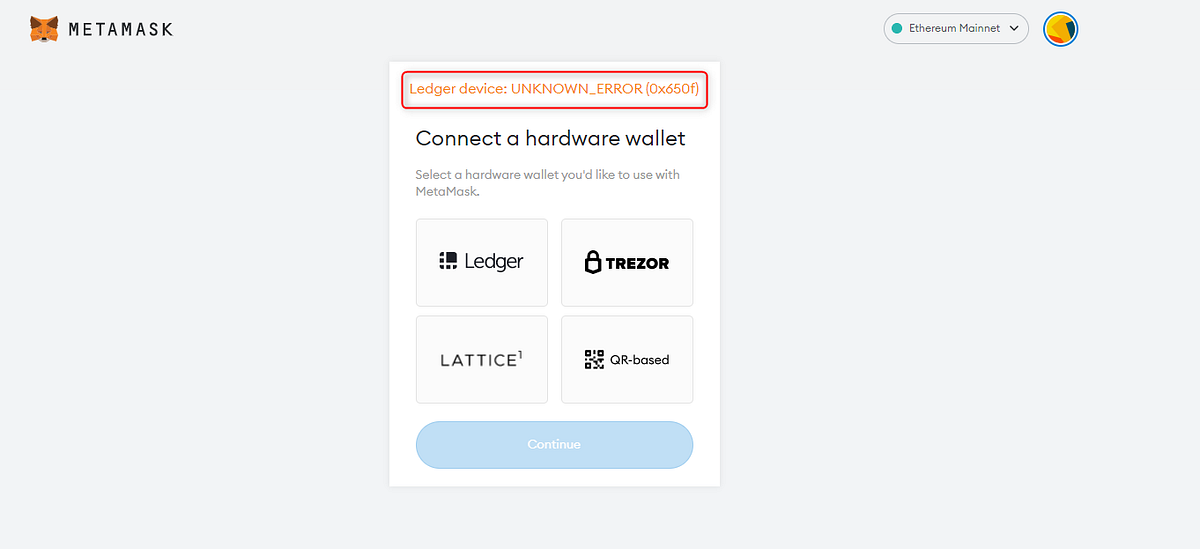The image depicts the MetaMask interface, prominently featuring a fox's face in the top left corner. In the top right, it displays "Ethereum Mainnet" alongside a small icon. Central to the image is a box labeled "Connect to Hardware Wallet," prompting users to select a hardware wallet to integrate with MetaMask. Available options include Ledger, Trezor, Lattice, or QR-based wallets. A notable error message appears at the top, reading "Ledger device unknown error 0x650F." This suggests an attempt to add a Ledger hardware wallet that resulted in an error. MetaMask is a tool used for managing cryptocurrency, and hardware wallets like Ledger provide an added layer of security.